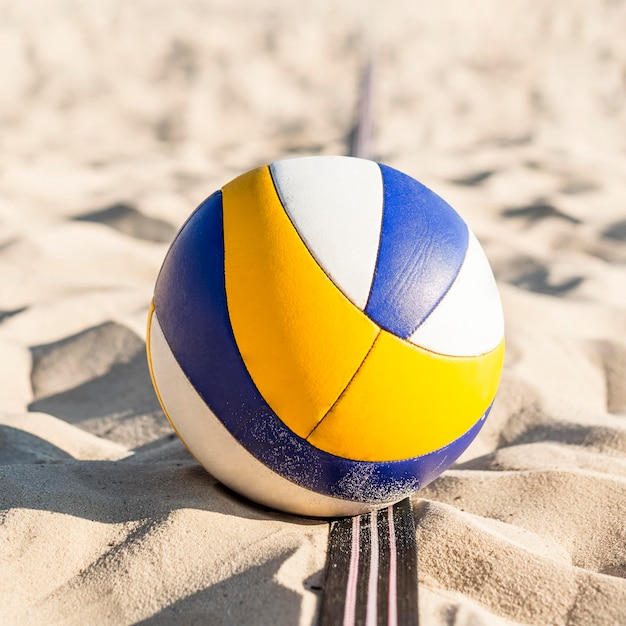This detailed photograph captures a vibrant and lively beach scene with the focal point being a white ball adorned with blue and yellow stripes, characteristic of a volleyball. The ball rests on light brown sand, partly covered in grains, signifying its interaction with the beach surface. Prominently in the foreground, extending from the bottom center and tapering off into the blur of the background, lies a conspicuous black strap embellished with three white stripes. This strap might be part of the sporting setup, possibly delineating the boundary of a volleyball court. The bottom of the photograph is sharply in focus, highlighting the ball and the strap, while the upper portion becomes progressively blurry, enhancing the depth of field. The outdoor daytime lighting creates shadows cast to the left, indicating the sun is positioned towards the right side of the frame, enriching the texture and contrast of the sandy beach environment.